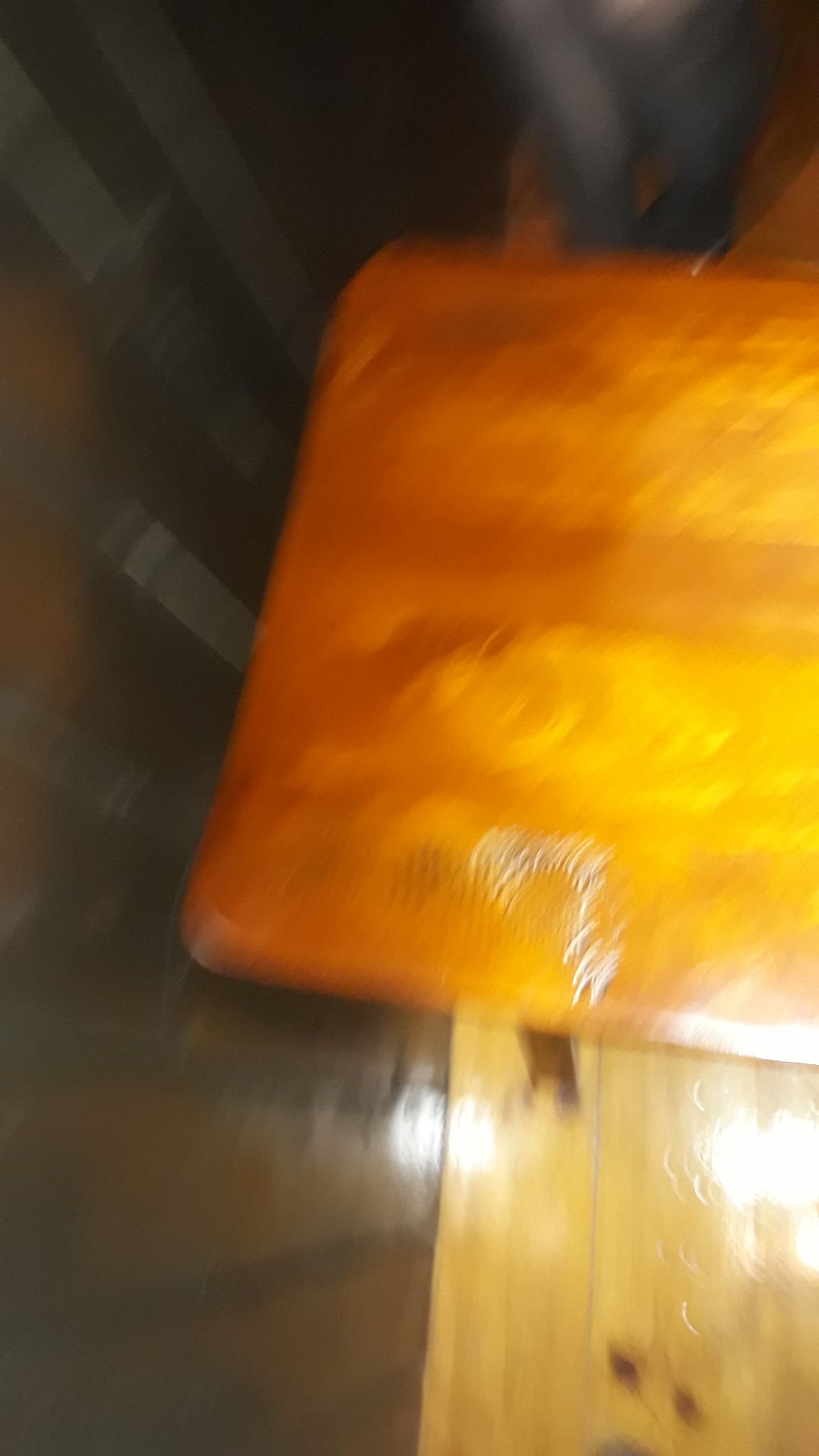An image depicting a blurry and out-of-focus scene, likely caused by camera movement or a bump. Dominating the background is a wood grain surface, indicative of a blonde wood floor, leading towards the corner of a room. On the left side, the wall seems to draw nearer as the floor extends towards the viewer's perspective. Central in the image sits an orange-striped square object, slightly elevated off the floor. This object might be a cushion, potentially the seat of a bar stool or another type of chair. Near the top of the image, what appears to be a structural component—possibly a leg or strut—rises from this cushion, further supporting the bar stool theory. Although the image lacks sharpness, the elements suggest a casual indoor setting focused on a piece of furniture.